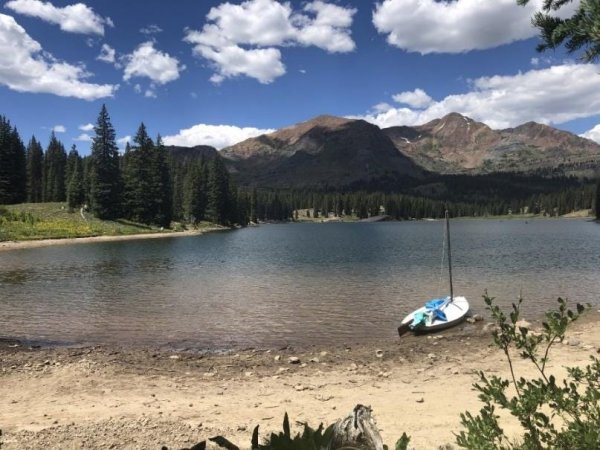In this picturesque outdoor scene, a small white sailboat is docked near the edge of a clear body of water, appearing in the bottom right quadrant of the image but not fully to the corner. Blue and teal garments lie on the boat's deck. The water reflects the blue sky and white clouds above, adding a serene touch to the scene. Towards the bottom and front of the image, a grayish-brown dirt beach is visible, interspersed with patches of foliage in the middle and lower right areas. 

Beyond the water, a grassy area with some tall trees stands to the left, transitioning into a backdrop of mountains. The mountains present a mix of barren brown peaks with less greenery, contrasting with the lush evergreens that grow densely in some spots and sparser in others near the water's edge. The sunlight illuminates the higher mountain peaks, casting shadows over the lower areas, underlining the landscape's varied textures and colors.